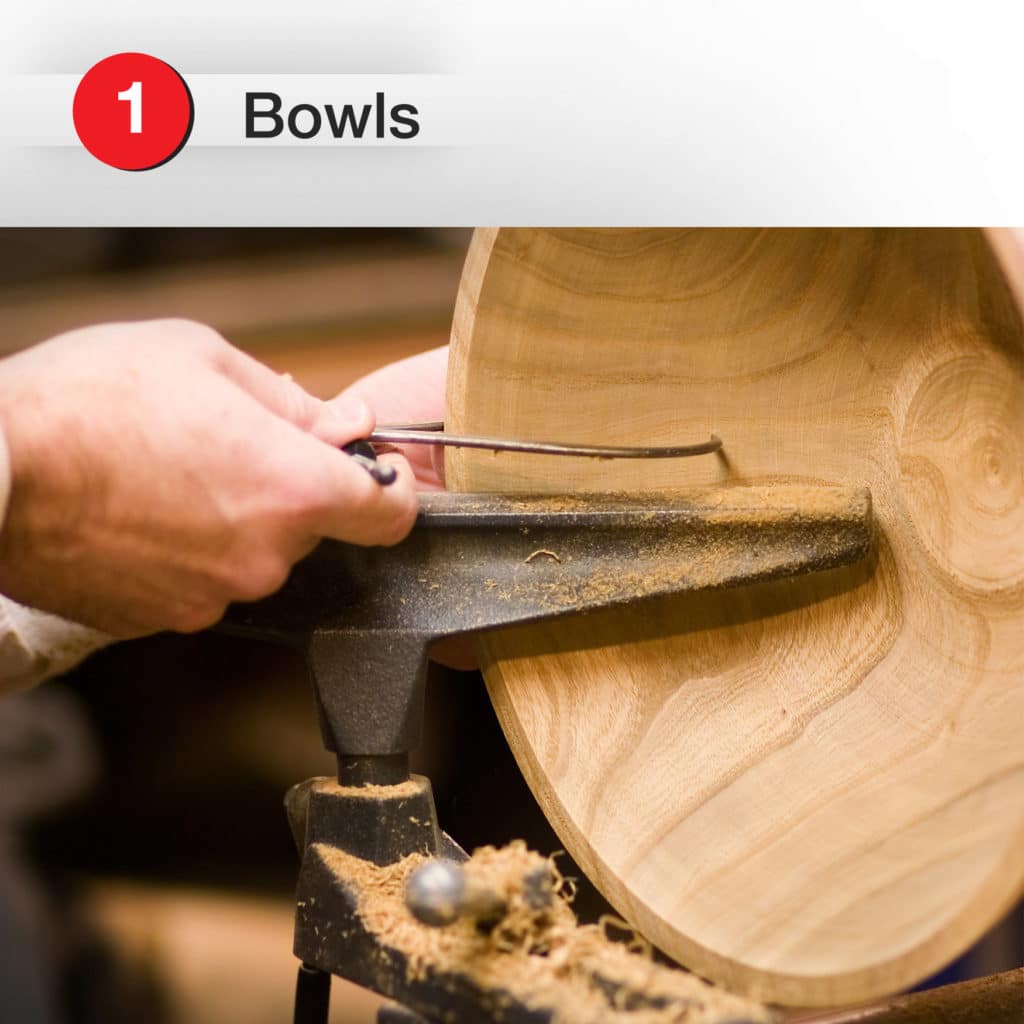This detailed image shows a skilled craftsman creating a light beige, wooden bowl on a spinning lathe. At the top of the image, a light gray rectangular banner extends across, displaying a prominent red circle with the white number "1" in it, accompanied by the word "bowls" in black print. The bowl itself is securely held in place by a central vice-like mechanism, with wood shavings visible in the lower center, indicating active craftsmanship. In the upper left section of the picture, a pale, male hand extends from the left, holding a thin metal tool, which is making precise cuts on the inside of the bowl. The crafting tool looks similar to an ice scraper but is designed for woodworking, highlighting the detailed, hands-on process of handmade bowl creation.